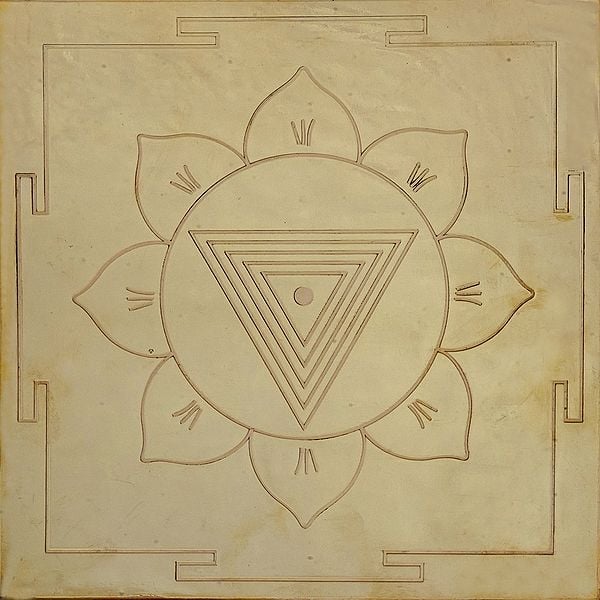The image depicts a detailed and intricate design with multiple layers and shapes, reminiscent of a divine yantra often used in Hindu rituals. The background appears to be a light, rusty-colored parchment or metal. At the center of the image is a large circle resembling a flower with eight petals radiating outward. Each petal features three vertical lines extending slightly outward.

Inside the circle, there are five concentric equilateral triangles nested within each other, all pointing downwards. At the very center of the smallest triangle, there is a small circular dot. Surrounding the large central circle is a square frame with flange-like extensions protruding from the middle of each side, creating a cross-like shape.

The entire design is detailed with lines slightly darker than the background, in shades of gray-brown, giving it a faded, almost ancient appearance. The overall composition creates a sense of symmetry and sacred geometry, typical of a yantra used for divine purposes, predictions, or rituals.